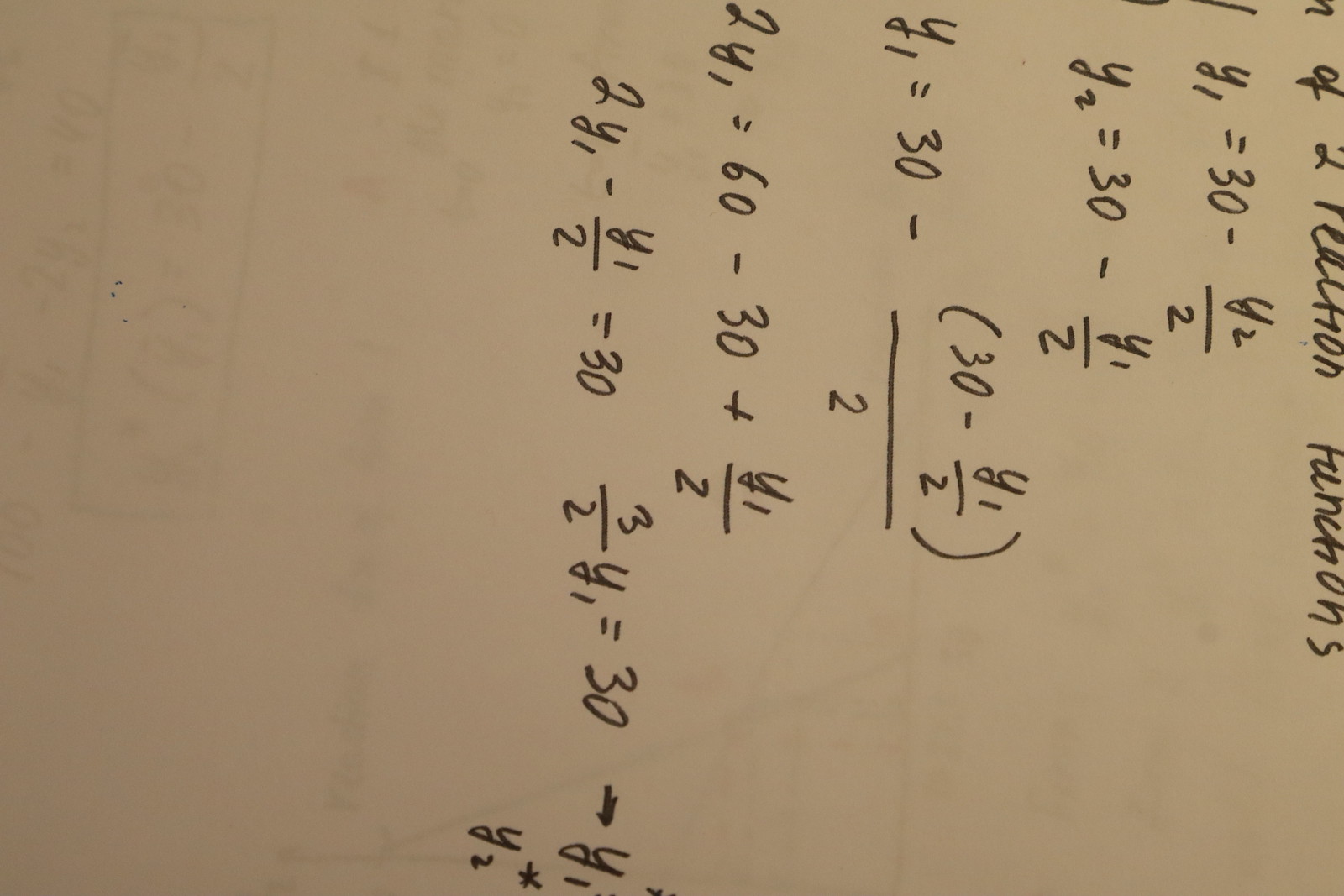A detailed caption for the given image:

"Photograph of a whiteboard with mathematical equations written in black marker. The whiteboard appears to be turned on its side, making the text difficult to read, and portions of the equations are clipped from the frame. The board itself looks light tan, though it is likely white with a color cast. The visible equations include a series of reaction (or possibly relation) functions and subsequent steps. The first equation reads 'y₁ = 30 - y₂ / 2,' followed by 'y₂ = 30 - y₁ / 2.' Further down, a more complex expression can be partially deciphered: 'y₁ = 30 - (30 - y₁ / 2) / 2,' evolving into '2y₁ = 60 - 30 + y₁ / 2,' and '2y₁ - y₁ / 2 = 30,' leading to '3/2 y₁ = 30,' before getting cut off. The incomplete visibility of the text and side orientation add complexity to interpreting the equations accurately."